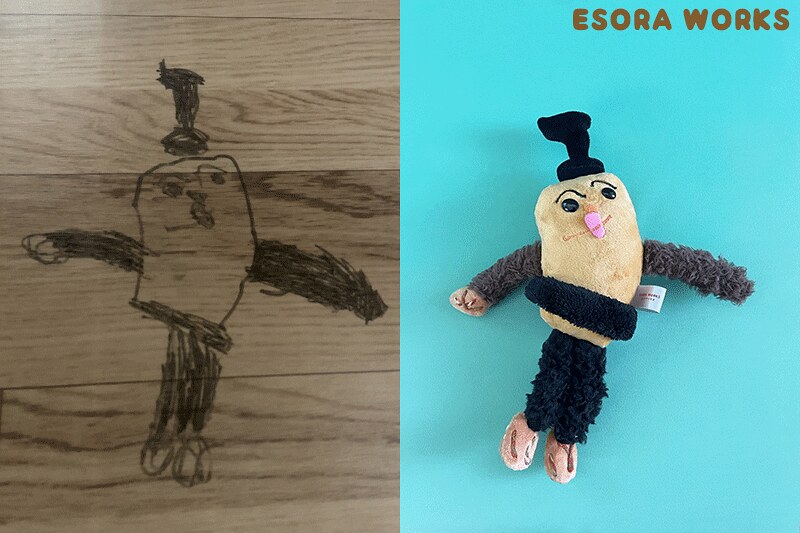The image features two distinct pictures side by side. On the left, there's a detailed drawing set against a light wood background. The drawing displays a rectangular-bodied figure with black-colored arms and legs ending in circle feet. The figure has detailed facial features, including two eyes, two eyebrows, a triangle nose, and a circle mouth. Atop its head, it wears a unique hat characterized by a circular base, a tall piece above it, and an object on top. The right side of the image reveals a plush doll inspired by the drawing. The plush is set against a teal blue background with "Azora Works" written at the top in brown lettering. The doll sports an oddly constructed design with a curved black top hat, round black eyes, a line mouth with pink lips, and an orange nose. It has grayish fur sleeves with visible fingers on the left hand and a light brown furry torso. A black band encircles its waist, and it has dark blue fur covering the lower body and light pink feet. The plush also features a fabric tag on its right side, precisely capturing the essence of the whimsical drawing on the left.